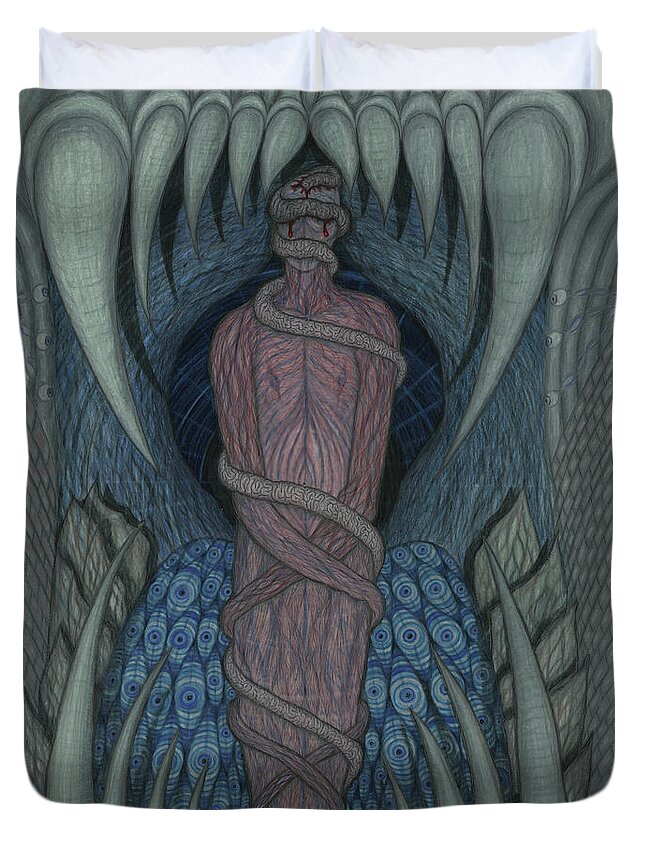This image showcases a dark fantasy-themed bedspread that melds disturbing horror elements and vividly grotesque artistry. Set against a plain white background, we see a bed arranged with two white pillows at the top. The bedspread itself appears to be a product photo designed for an online marketplace where users can sell custom-printed items like on Cafe Press.

Dominating the scene is the blanket that portrays a menacing, open mouth filled with sharp, grayish-green fangs, suggesting an otherworldly creature. The interior of the mouth reveals a sinister blue tongue, patterned with elongated circles and swirls, creating a chilling visual effect. At the center of this mouth, bound in haunting detail, is a humanoid figure rendered in stark, skinless maroon hues, highlighting exposed musculature. The figure's arms are crossed and entwined in vine-like, snake-like tendrils that coil around the body, spiraling upward.

These tendrils appear to merge into serpents or intestines, wrapping around the head-like form and piercing its skull, from which blood seems to ooze. This grotesque imagery evokes the aesthetic of a death metal album cover, presenting a nightmarishly intricate design that pushes the boundaries of dark fantasy art into the realm of surreal horror.